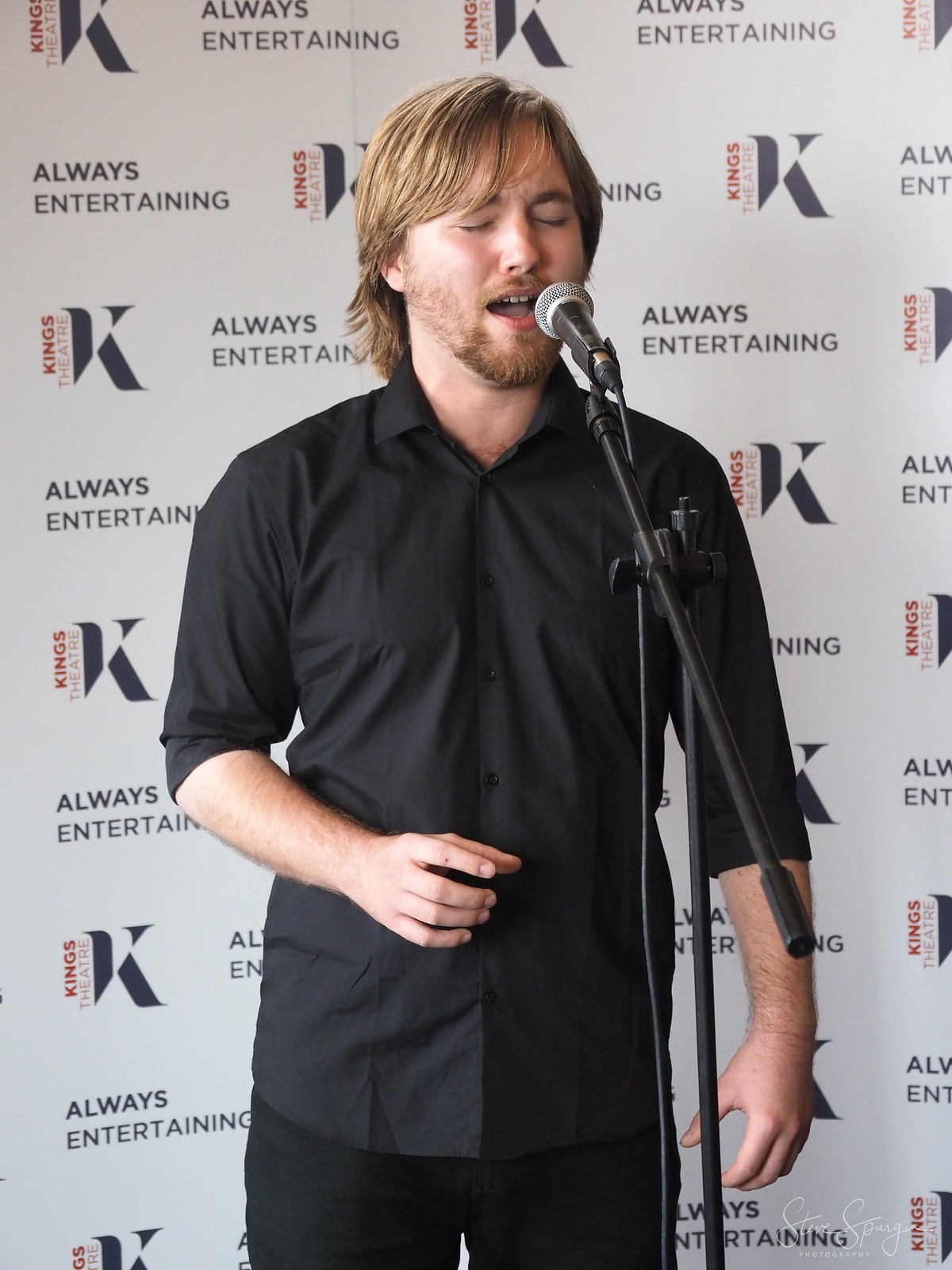A man stands at a microphone, positioned at his face level, with one hand raised and gesturing while he sings, and the other hanging by his side. He has light brown, sandy-colored hair that partly covers his eyes and ears, and he sports a beard and a mustache. Dressed in black formal attire, including a collared button-up shirt and black pants, he exudes a serious and professional demeanor. His shirt sleeves are rolled up just below his elbows. Behind him is a prominent white banner adorned with repeated text in black: "Always Entertaining," interspersed with the red and gold logo of the King's Theater, which features a large "K" and the words "King's Theater" arranged vertically. In the bottom right corner of the image, the cursive signature "Steve Photography" can barely be deciphered, attributing the photograph.